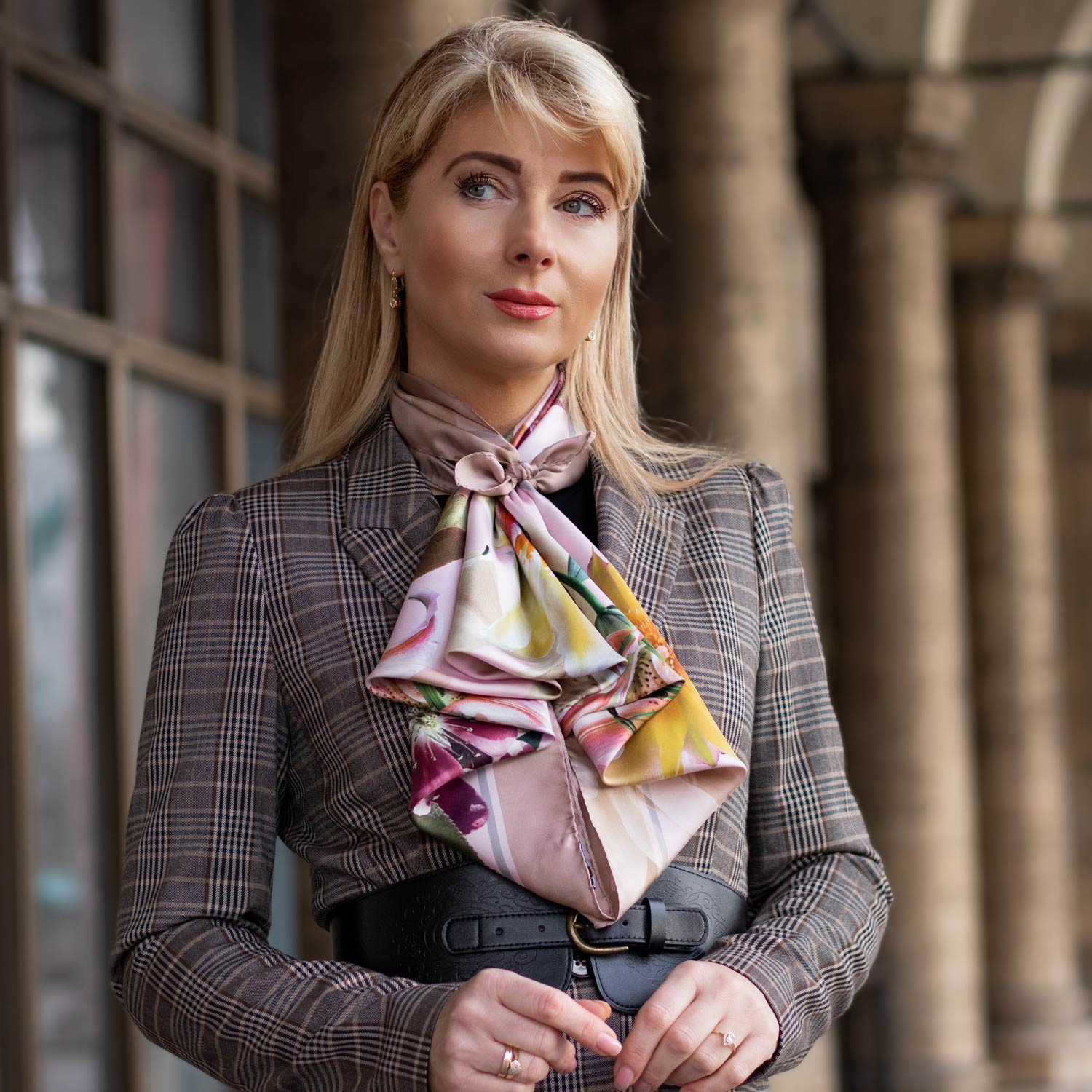The image features a blonde-haired, white woman in her 30s or 40s, who exudes a professional and put-together appearance. She wears light pink lipstick and has well-done makeup, enhancing her perfect complexion. Her darkly painted eyebrows accentuate her light blue eyes, which gaze slightly upward to her right, although she faces forward.

Her outfit is a harmonious blend of prints and textures. She sports a large, floral-patterned scarf that is dramatically tied into a bow at her neck before cascading down to cover her chest. Over this, she dons a plaid flannel business suit jacket, featuring a mix of brown, white, and black tones, detailed with long sleeves and neatly fitting hands. Around her waist is a distinctive black belt, reminiscent of a back support brace, securing tightly with an additional conventional belt.

Accessorizing her ensemble further, she wears rings on both hands, including a notable ring on her right index finger. In the background, the architectural setting includes three marble arches visible over her left shoulder and large windows framed by columns over her right shoulder. She stands confidently, with a radiant smile, embodying poise and elegance.